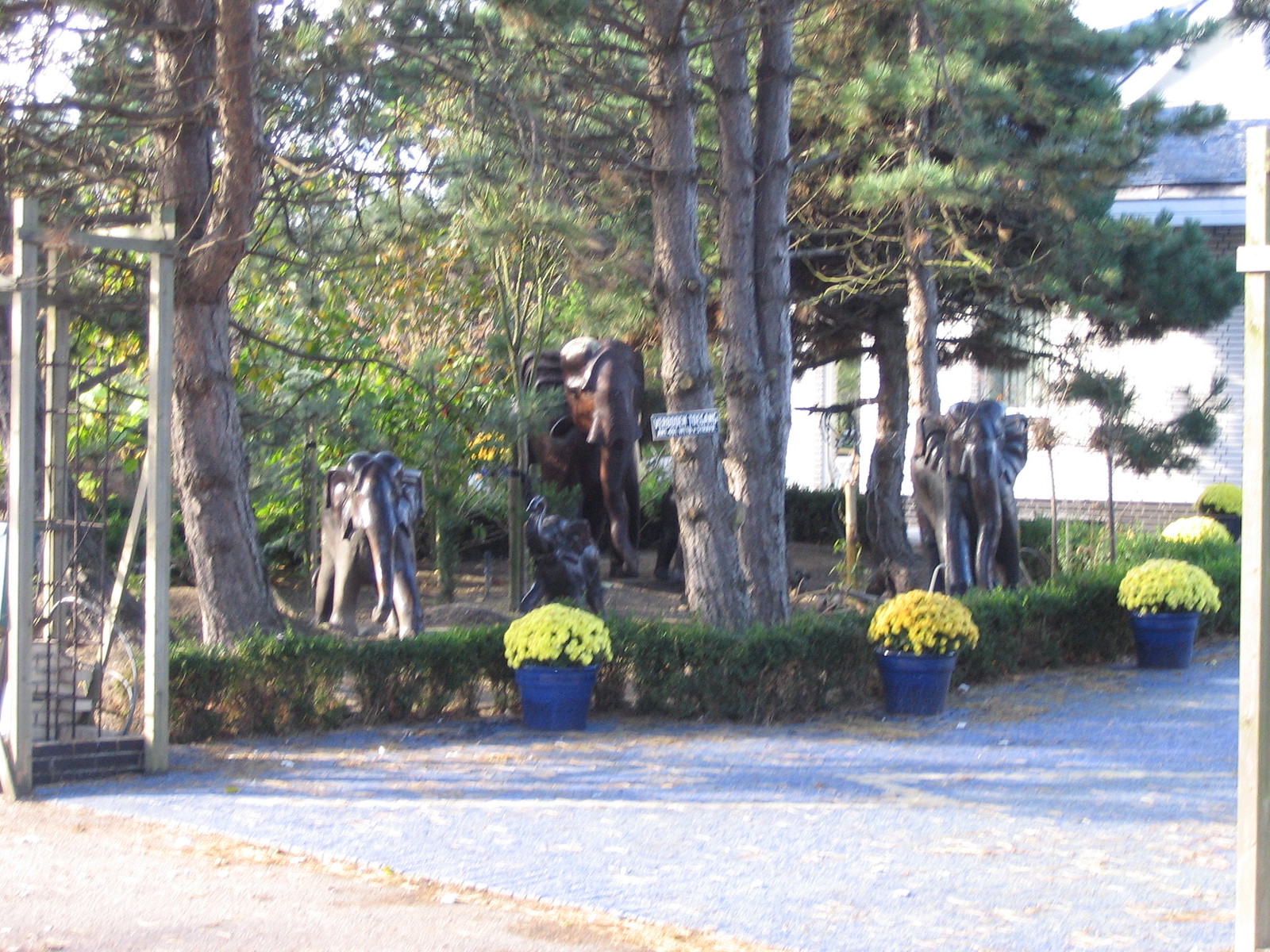The image portrays a faded, slightly overexposed color photograph that appears to have been taken outdoors in a park or garden. The photograph, itself a snapshot, features a small white border and a few clips on the right-hand side, indicating it was perhaps pinned down and re-photographed. Dominating the scene are several tall evergreen trees, likely pine or hemlock, with their lower branches trimmed off. Beneath these trees, there are a series of stone statues, including at least four elephants—two smaller gray ones on the ends and a larger brown one in the middle. The elephants are arranged with their heads facing outward towards the viewer.

In the foreground, a low green hedge runs diagonally across the scene, separating a gravel driveway from the area where the trees and statues are situated. Along the edge of the hedge are blue flower pots filled with vibrant yellow flowers. These planters extend from the center of the image towards the right-hand side. The background reveals a stone or stone-like white building, completing the picturesque garden setting under a bright and sunny sky.